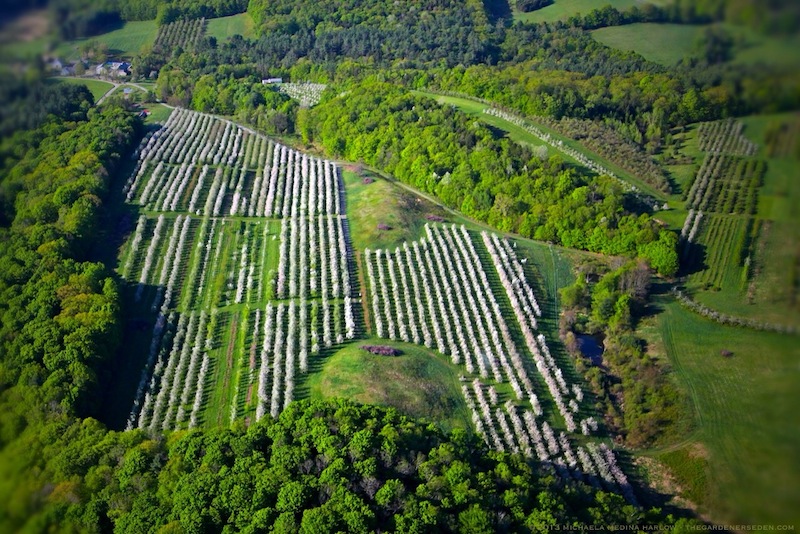This is an aerial photograph of a vast orchard field, displaying rows upon neatly aligned rows of large trees, likely fruit-bearing, interspersed with small man-made mounds disrupting the rows in the center of the top and bottom sections. A dirt road snakes through the landscape, running alongside the fields and leading to a cluster of buildings in the top left corner, which appear to be houses, garages, or warehouses. A distinct tree or hedge row separates an additional set of tree rows to the right of the field. The terrain features rolling hills and lush greenery, accentuated by a few barely discernible lines of white text in the bottom right corner. There's a hint of pastoral life with a small flock of sheep visible near the roadways, adding a touch of dynamic life to an otherwise serene agricultural expanse.